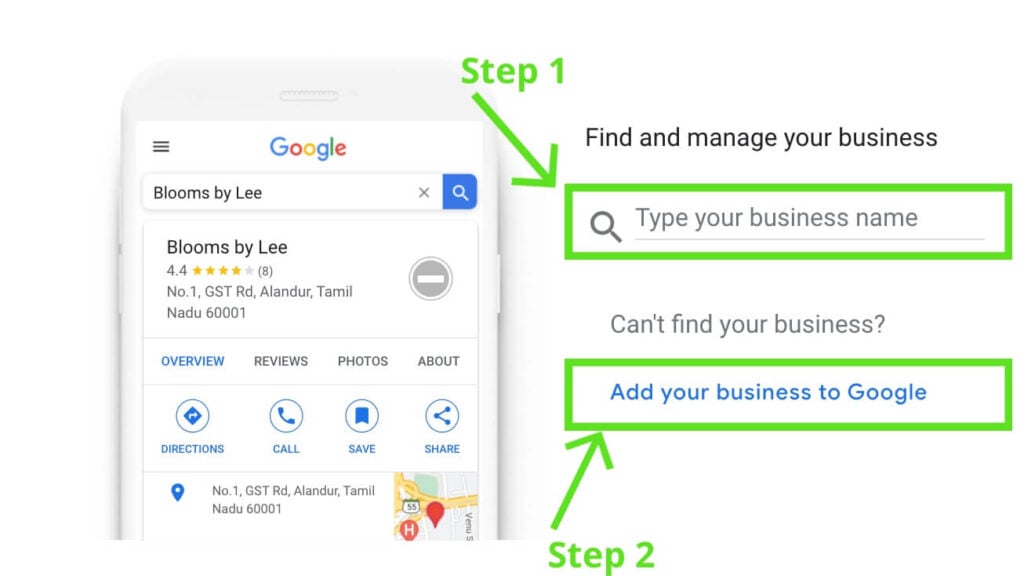"The image appears to be a screenshot from a computer, providing detailed instructions on how to find and manage a business via Google. On the left side of the image, there is a graphic representation of a smartphone with a white screen. At the top of the phone's screen, the colorful 'Google' logo is prominently displayed, followed by a search bar where 'Blooms by Lee' has been typed. The search results show 'Blooms by Lee' with an impressive rating of 4.4 stars, located at '1 GST Road, Allender to meal, 600001'. Underneath the address, various interactive options are presented in icons for 'Directions', 'Call', 'Save', and 'Share'. At the bottom, a small map and a location pin provide a visual reference of the business's location.

On the right side of the image, instructions are given for managing a business listing. The text at the top reads 'Find and manage your business,' followed by a prompt to 'Type your business name,' enclosed in a green rectangle with an arrow labeled 'Step 1' pointing towards it. Below this, there's a section that says 'Can't find your business?' followed by an option to 'Add your business to Google,' highlighted in blue with a green rectangle around it. Another arrow labeled 'Step 2' points towards this prompt, guiding the user through the process of adding their business to Google."